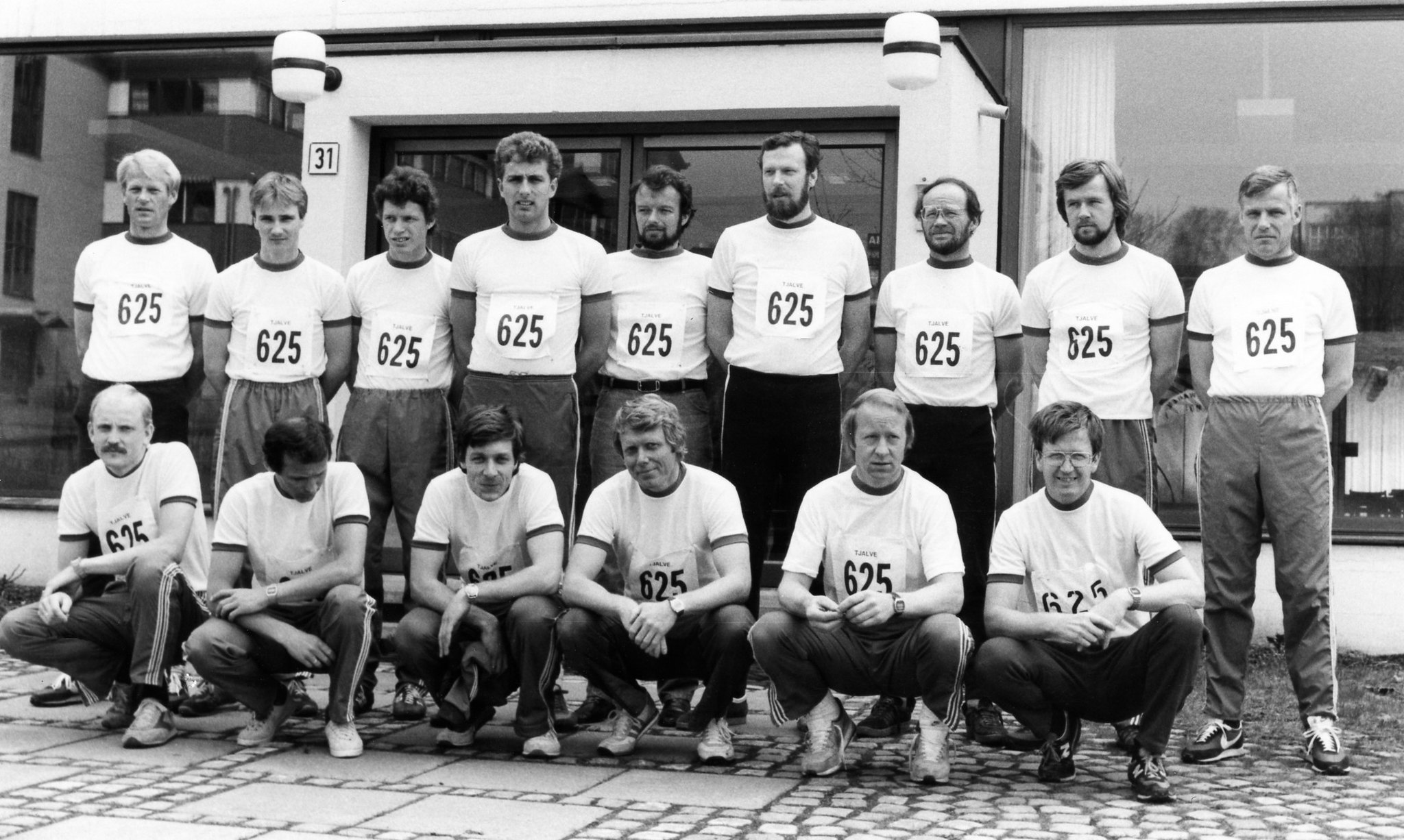This black and white photograph features a group of men, likely participating in a sports team event, gathered in two rows in front of a building with large glass windows and a sign labeled "31" to the left of the entrance. The group consists of 15 men, with 6 kneeling in the front row and 9 standing behind them. Each man is attired in a white shirt emblazoned with the number "625" and darker-colored pants, some of which have a stripe down the middle. Despite the photo's monochrome nature, the varying shades of the pants suggest that they are different colors. The men, who appear middle-aged, look towards the camera with some smiling. The scene is set on a cobbled or tiled surface, adding to the image's vintage feel. The overall setting and attire hint at a possible athletic context, such as a swimming, track, or soccer team.